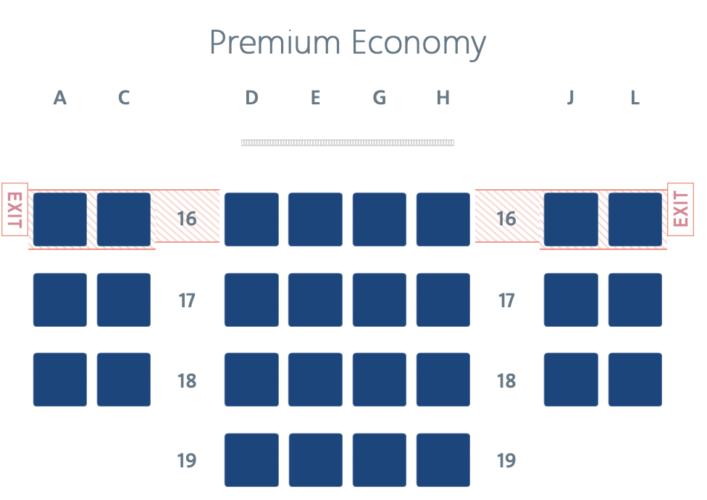The image depicts the layout of a premium economy section in a large aircraft, likely a jumbo jet, featuring a detailed seating arrangement for rows 16 through 19. The plane has two aisles, creating three distinct sections of seats: left, middle, and right. 

Row 16 is marked as an exit row, evident from the "EXIT" signs on both sides, highlighted by an orange lattice or fencing for clear visibility. In this row, all seats appear to be blocked, possibly due to increased legroom or emergency exit requirements.

Rows 17 and 18 each consist of eight seats: two on the left (labeled A and C), a middle section with four seats (labeled D, E, F, and G), and two on the right (labeled H and L). Row 19, however, only has the middle section with four seats (D, E, F, and G), without any seating on the far left or right. The layout is set against a white background, and each seat is represented by a blue box.

Additionally, the labeling convention skips certain letters; there are no seats labeled B or K, despite the far-left seats being labeled as A and the far-right as L, possibly due to airline-specific layout preferences or to avoid confusion.